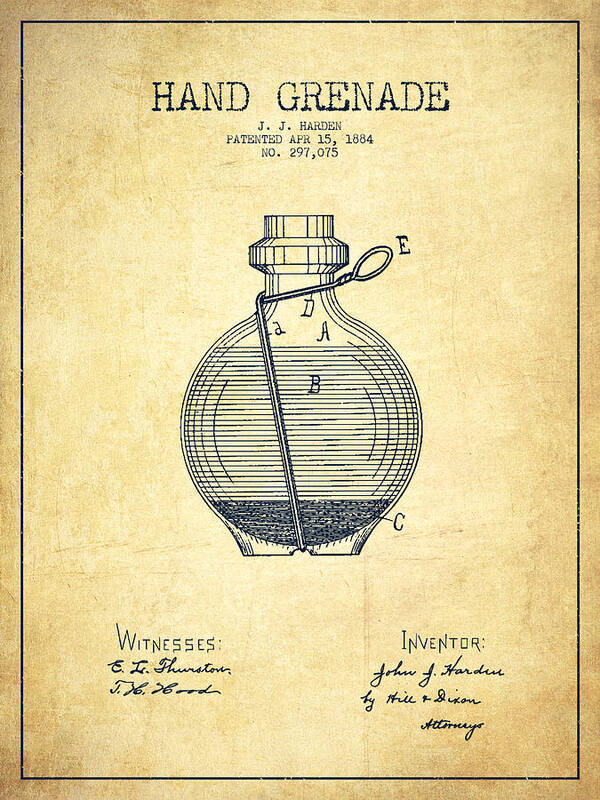The image depicts a detailed illustration of a vintage hand grenade on an old, brown, grainy sheet of paper, which has a yellowish hue and a square-like shape. The paper features a thin black line border framing the contents. At the very top of the sheet, in black letters, it reads: "Hand Grenade, J.J. Hardin, Patented April 15, 1884, No. 297,075." Below this text is a technical diagram of the hand grenade, showcasing a bulbous body that transitions into a neck area. Around the neck, a metal wire is intricately looped, extending to the right, down across the body, and terminating at the middle bottom part of the grenade. The diagram also includes the letter "E" on the top right of the grenade and the letter "C" on the bottom right, while the word "Witnesses" is inscribed on the bottom left. The overall artwork and text are rendered in black, contributing to the antique and technical appearance of the document.